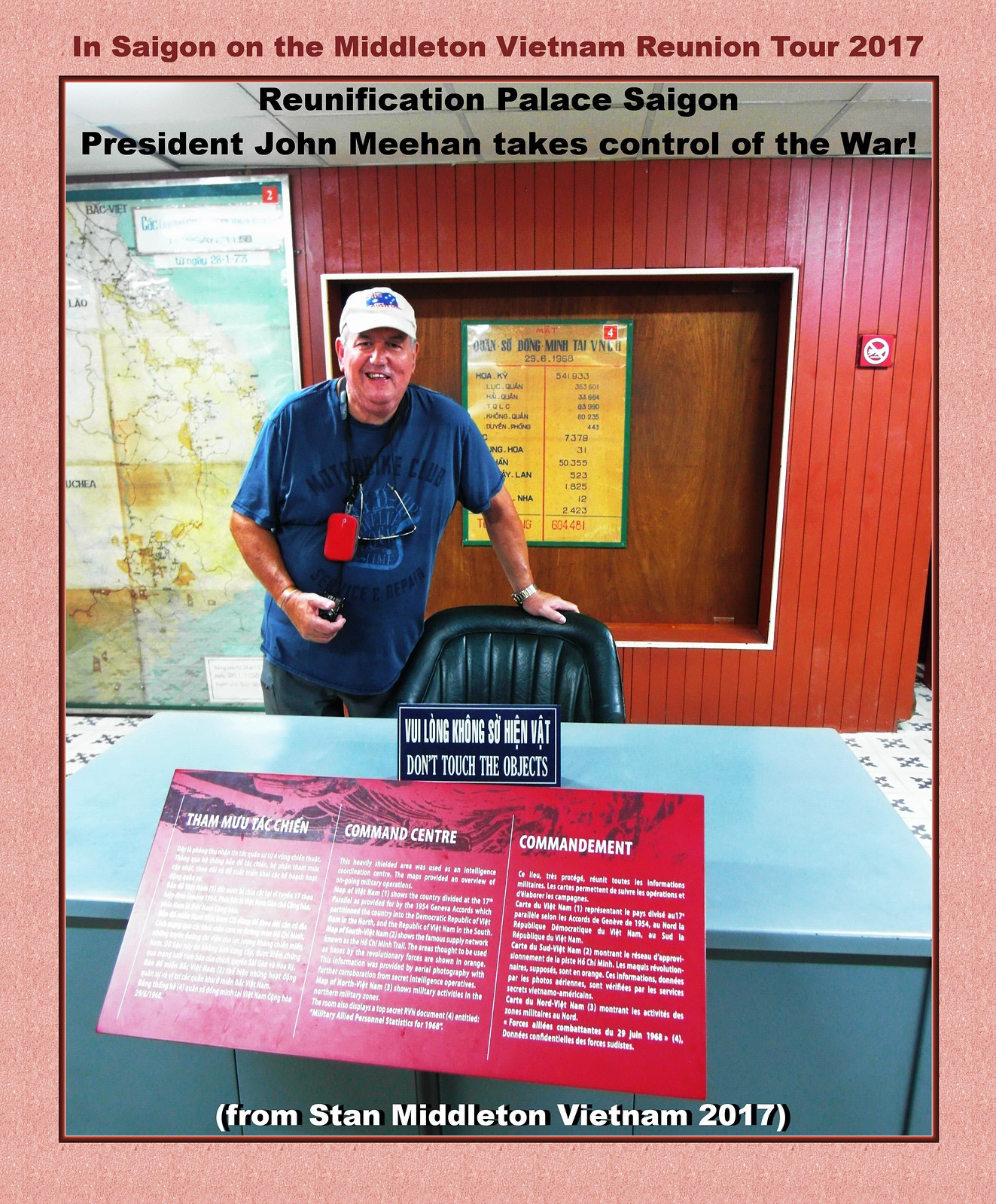The image features a detailed photograph inside a room, bordered by a distinctive red frame. At the top, the text reads, "In Saigon on the Middleton Vietnam Reunion Tour 2017." Central to the photograph is an inscription, "Reunification Palace Saigon, President John Meehan takes control of the war." A man, wearing a white baseball hat with a graphic, a blue t-shirt, blue jeans, and with glasses hanging from his neck, stands prominently. He is positioned behind a black leather chair next to a blue desk. The desk prominently displays a sign that says, "Do not touch the object." Behind the man, a large map is visible on the left, while the background includes an indiscernible poster on the wall. Below the photograph, it reads, "From Stan Middleton, Vietnam 2017." The entire image is framed by a light pink-salmon colored border with dark red text, adding to its distinctive visual context.